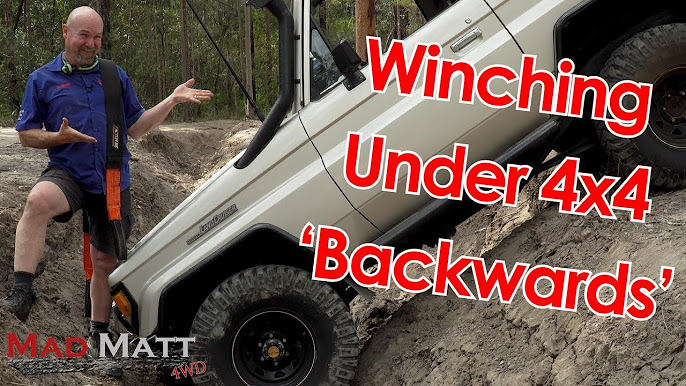The image depicts a bald Caucasian man, identified as "Mad Matt" from his YouTube channel "Mad Matt 4WD," standing and gesturing towards a Land Cruiser 4x4, which is being winched backwards out of a muddy ditch in a camping area surrounded by trees. Mad Matt, a 4x4 enthusiast who possibly creates content on vehicle recovery techniques, is smiling and dressed in black shorts, black boots, and a blue button-up shirt. The Land Cruiser is tilted forward into the ditch with no one inside, and the scene is accentuated by a caption that includes the words "winching under 4x4 backwards" in quotations at the bottom left corner.